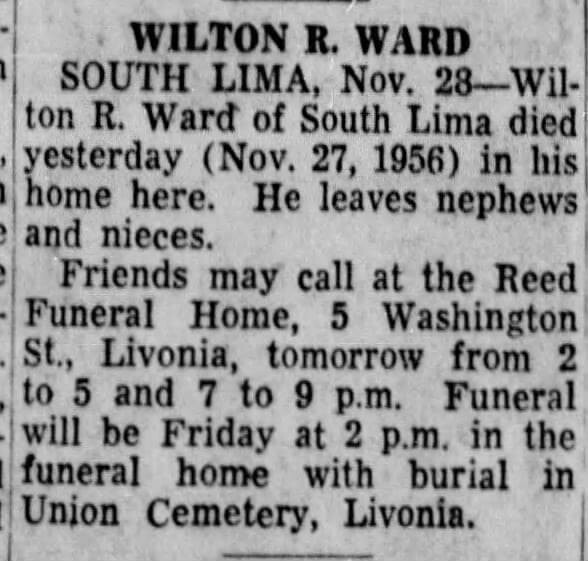The image captures a close-up scan of a cropped obituary from a newspaper, set against a white background with black text. At the top of the obituary, in bold and capitalized letters, is the name "Wilton R. Ward." Directly underneath, it states "South Lima" in all caps, followed by the date "November 28." The text continues to convey that Wilton R. Ward, of South Lima, died on November 27, 1956, in his home. He is survived by nieces and nephews. The obituary informs that friends may call at the Reed Funeral Home, located at 5 Washington Street, Livonia, tomorrow from 2 to 5 p.m. and 7 to 9 p.m. The funeral service is scheduled to be held at the funeral home on Friday at 2 p.m., with burial to follow in Union Cemetery, Livonia.